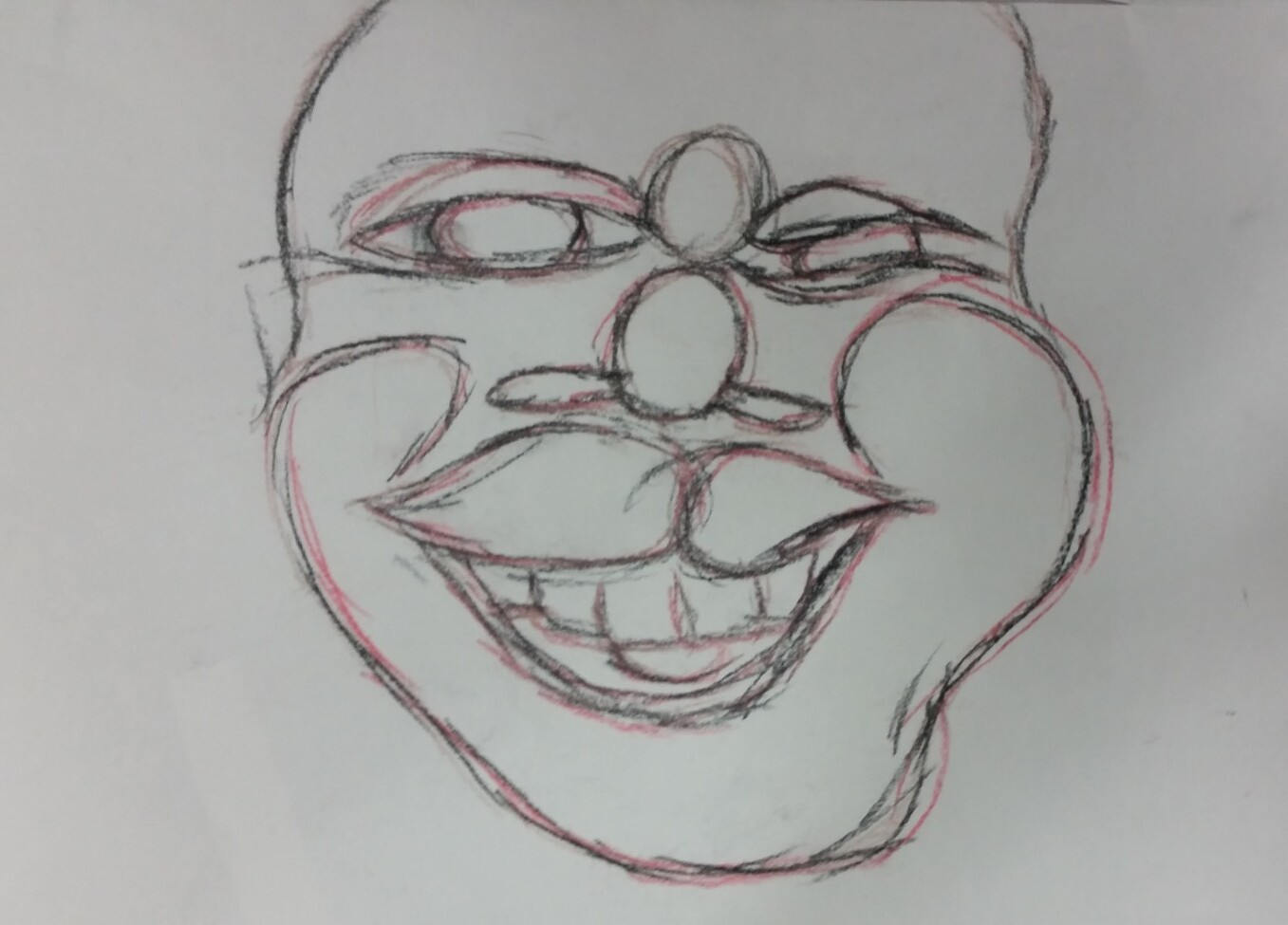The image features a sketch of a bald man's face centered against a medium dark gray background with a width approximately 30% greater than its height. The sketch, rendered in overlapping black and red colored pencil lines, portrays a chubby face with pronounced rounded features reminiscent of a clown. The eyes are depicted as narrow slits, giving a glimpse of the circular pupils, and are topped with eyebrows. Between the eyes, a small circular mark is visible, just above another circle representing the nose. The nose features two rounded extensions at either side. A distinctive mustache, shaped like intersecting horizontal raindrops with their wider ends meeting at the center, adorns the face. The man sports a wide smile revealing large, square front teeth and a tongue, framed by big, rounded, rosy cheeks.